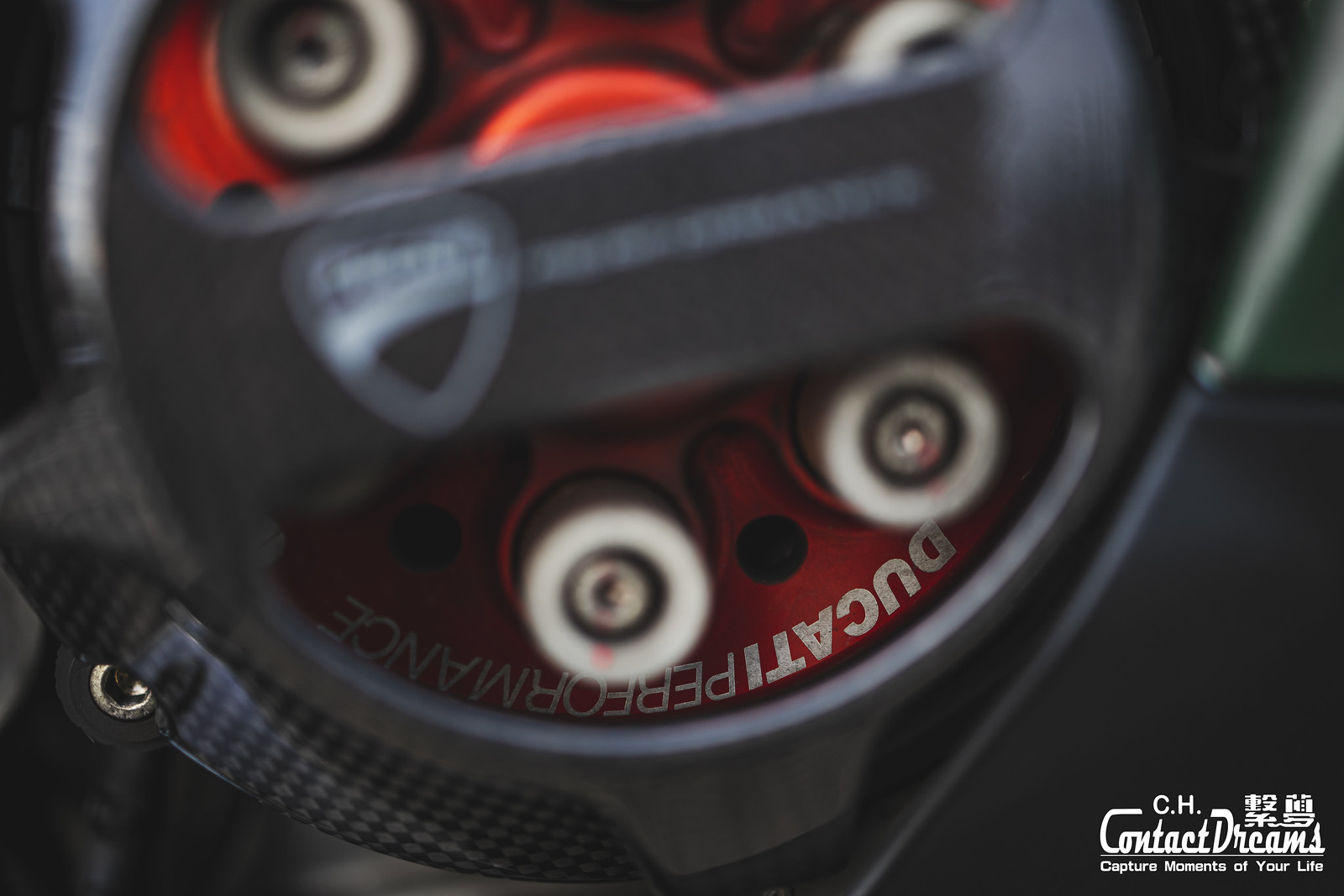The photograph features a professionally taken, close-up image of a motorbike part, most likely associated with Ducati due to the clearly visible text "Ducati Performance" prominently displayed on a red section of the part. This macro-style shot is sharp and focuses on the text while slightly blurring the background. The part appears to be a cylindrical object with a black exterior, containing a red cylinder inside it. Within this red section, there are four white cylindrical items, resembling batteries or small metal components, each capped in silver and standing on end. The black and red contrast highlights the text and gives a sleek, mechanical appearance. In the bottom right corner, there is a white watermark for "CH Contact Dreams," along with their tagline "capture moments of your life," and accompanied by a few Chinese characters, indicating either the photographer or the company protecting the image. Overall, the image suggests a high-quality product or component, possibly part of an advertisement.